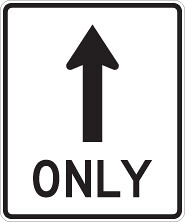This digital illustration showcases a small, rectangular white sign with a slightly rounded black border and corners. The sign features an upward-pointing black arrow centered in the upper portion, followed by the word "ONLY" in bold, uppercase black text situated at the bottom. Surrounding the main body of the sign is a very thin, barely noticeable black trim that adds a subtle touch to the frame. The entire sign is set against a plain white background, emphasizing its simple yet clear directive: "UP ONLY."